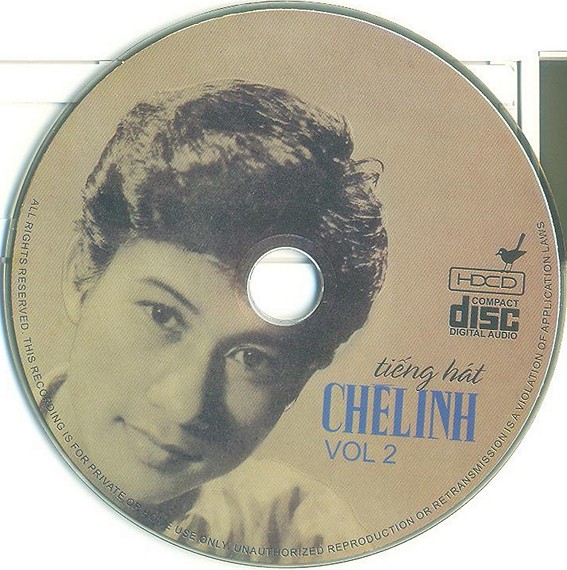The image depicts a CD with a light brown to tan background. At the center of the CD, there is a black and white image of a male with medium-length brown hair, slightly styled back. The male's head is tilted towards the left and the center hole of the CD aligns with the middle of his forehead. Written prominently on the CD is the title "Tinh Hat," followed by "Che Linh, Volume 2" in blue letters.

Above the text, there is a small black bird perched on top of the "HDCD, compact disc, digital audio" logo. Around the bottom perimeter of the CD, there is faint text stating legal information: "All rights reserved. This recording is for private or home use only. Unauthorized reproduction or retransmission is a violation of applicable laws."